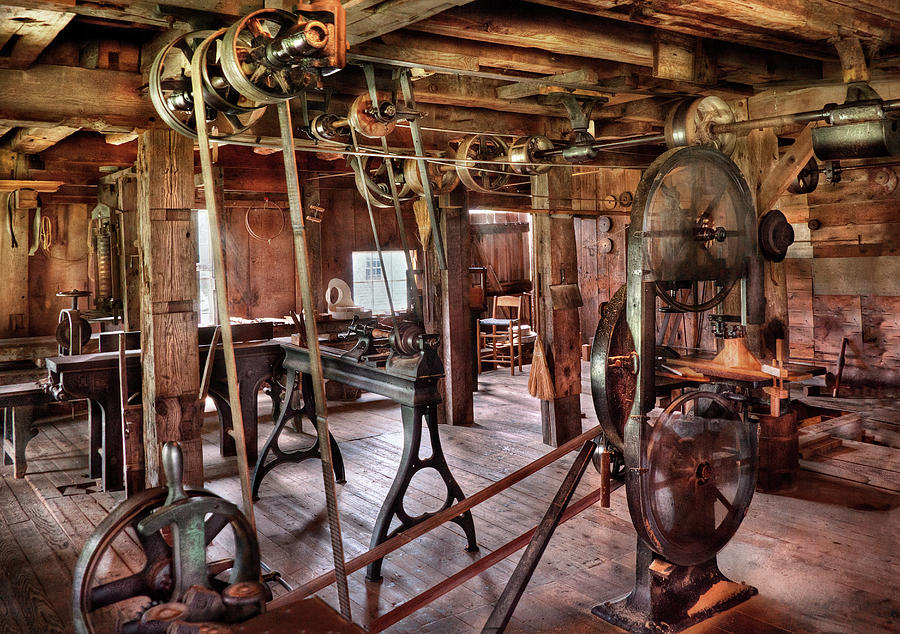The image depicts the interior of a historical workshop, giving the impression of an 1800s era setting. The entire structure, including walls, ceiling, floors, and support beams, is crafted from richly detailed dark brown wood. Numerous large, cast iron and mechanical machines are scattered throughout the workshop, some featuring spinning gears and belt-driven wheels. These antique machines could be used for woodworking, sewing, printing, or bookbinding, indicating a versatile yet ancient manufacturing space. The atmosphere is further characterized by small windows towards the back, wooden poles that support the building, and visible sawdust near a wooden clamp, hinting at the once-active nature of this now abandoned and meticulously preserved space. There are no people present, emphasizing the workshop's antiquated and historical nature.